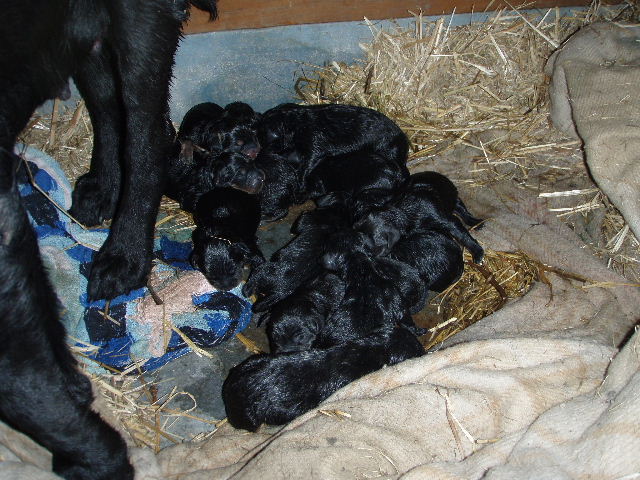This color photograph depicts a tender scene of a mother dog and her newborn puppies in what appears to be an outdoor barn area. The central focus is on a huddle of 11 or 12 tiny, shiny, black puppies nestled closely together, likely sleeping. Their uniform black fur makes it challenging to distinguish individual details, though a few show subtle brown markings on their faces. They lie on a mix of light blue, grayish, and tan blankets, surrounded by yellowish-gray hay, suggesting the puppies are in a cozy but rustic environment.

To the left, partially cropped from the frame, stands the mother dog, also black and with slightly damp-looking fur, indicating a recent birth. Only her hind legs, part of her stomach, and portion of her left leg are visible as she stands on a blue-patterned towel. The image captures the tender beginnings of these little puppies, enveloped in a setting that underscores the simplicity and raw beauty of new life.